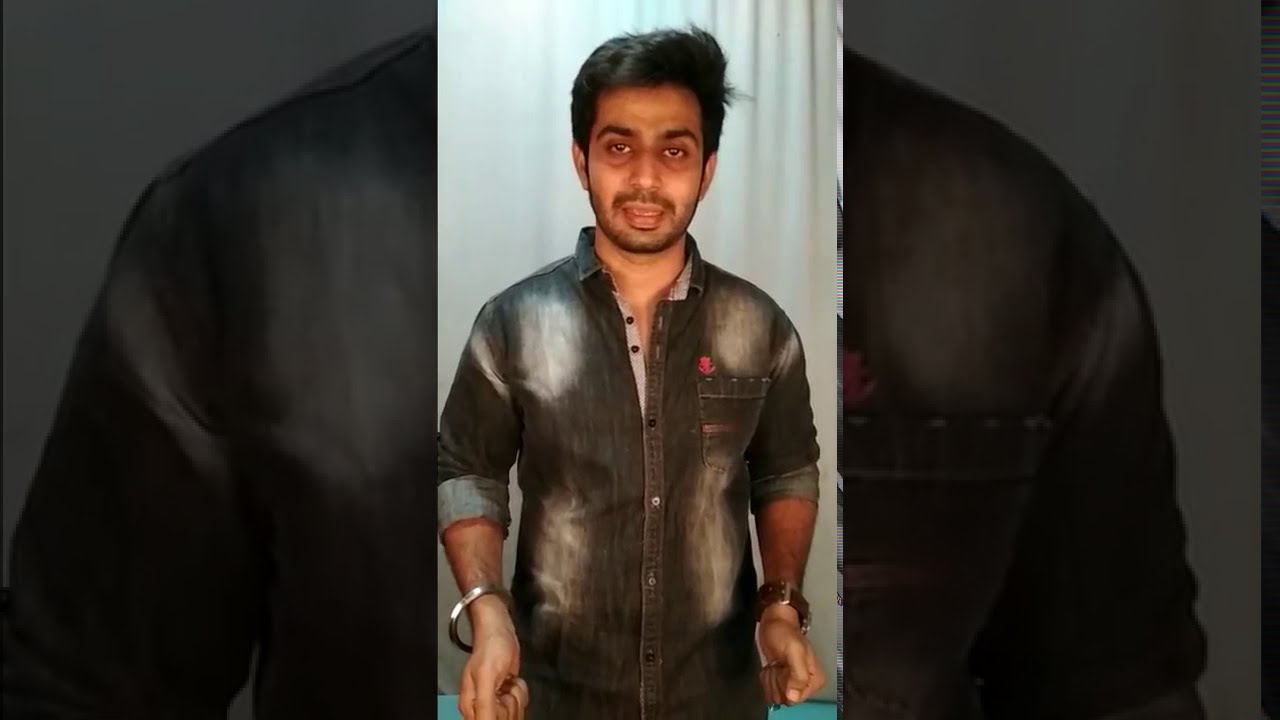This portrait-style image features an Indian man with tan brownish skin, black hair parted to the side, and a closely shaven black beard and mustache. He is depicted from the head to the top half of his torso, set against a white curtain backdrop with a light bluish-green floor. His expression suggests he is mid-sentence, with his mouth slightly open and looking directly at the camera. The man's hands, positioned by his waist, appear to be about to gesture, with his fingers clenched in fists. He wears a dark gray shirt with light patches on the shoulders, arms, and lower torso, along with a noticeable red flower above the pocket. His sleeves are rolled up, revealing a silver bracelet on his right wrist and a watch on his left. Some subtle details around his eyes imply he might be tired or have dark circles, adding depth to his face.